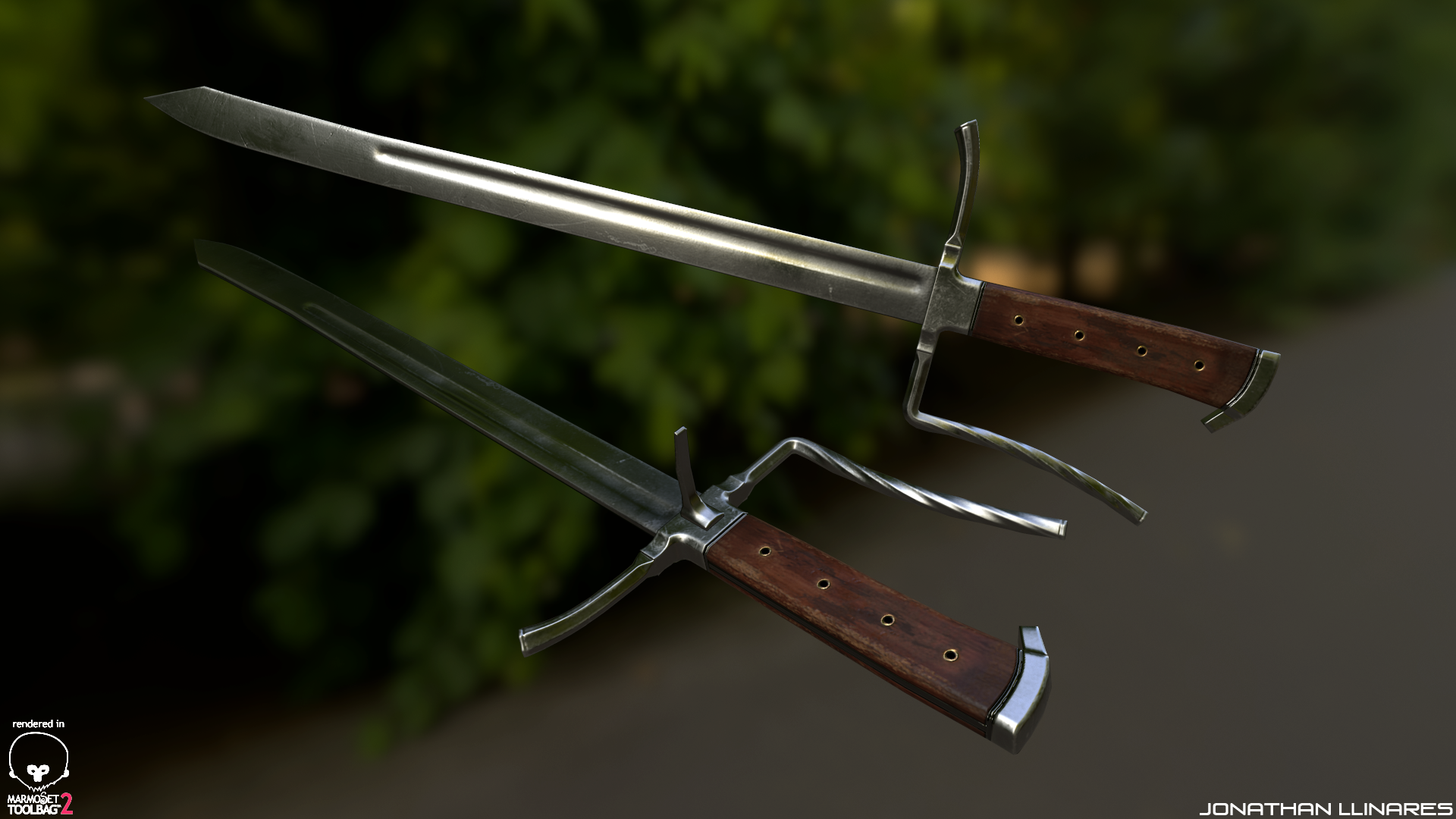This image is a digitally manipulated photograph featuring two knives or long daggers, appearing to float mid-air over a street scene background. Each knife has a brown wooden handle with four rivets and a silver-tipped pommel. The handles also include an upside-down L-shaped silver handguard that juts out at different angles, designed to prevent the hand from slipping. Both blades are short and pointed, with the knife on the left being slightly shorter than the one on the right. They are positioned with their blades pointing towards the upper left corner of the image.

In the blurred background, one can see a grayish sidewalk and green bushes. The photograph is signed by Jonathan Linares in the bottom right corner. Additionally, in the bottom left corner, there's a logo resembling a monkey with an afro and some writing indicating "rendered in marmoset tool bag 2" in pink.